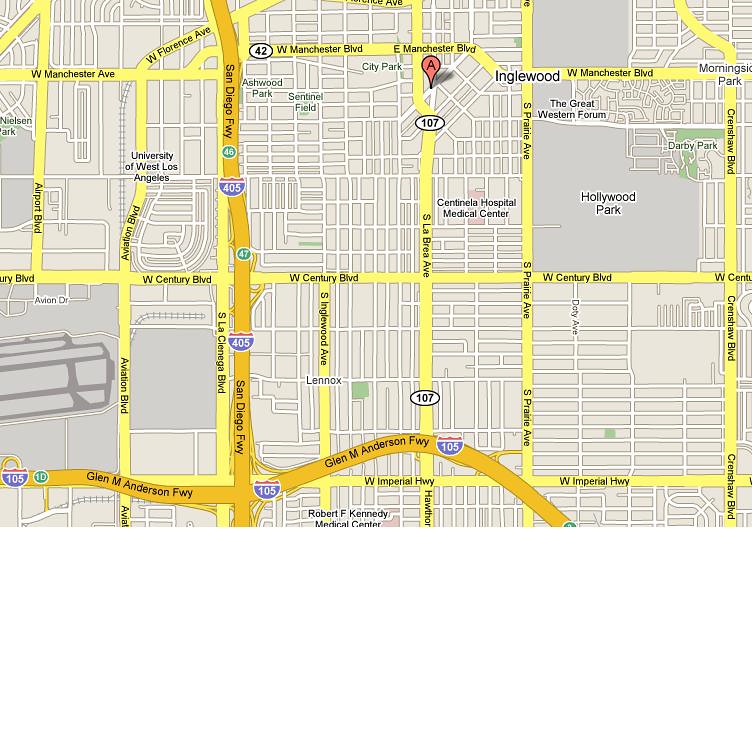This map features a gray background with streets highlighted in yellow and major roads in a yellowish-orange hue. The map is densely populated with text identifying various roads and highways. The main thoroughfare depicted is the San Diego Freeway, which runs vertically along the left side of the image. At the bottom, this freeway transitions to a horizontal orientation, intersecting with the Glenn M. Anderson Freeway, which extends from the left side of the map nearly to the right before veering downward and off the page.

Key roads at the top of the map include West Manchester Avenue, West Manchester Boulevard, and another segment of West Manchester Boulevard further to the right. Central to the image is West Century Boulevard, while towards the bottom, West Imperial Highway is prominently labeled. The detailed representation of these roads offers a comprehensive view of the area’s major routes and intersections.